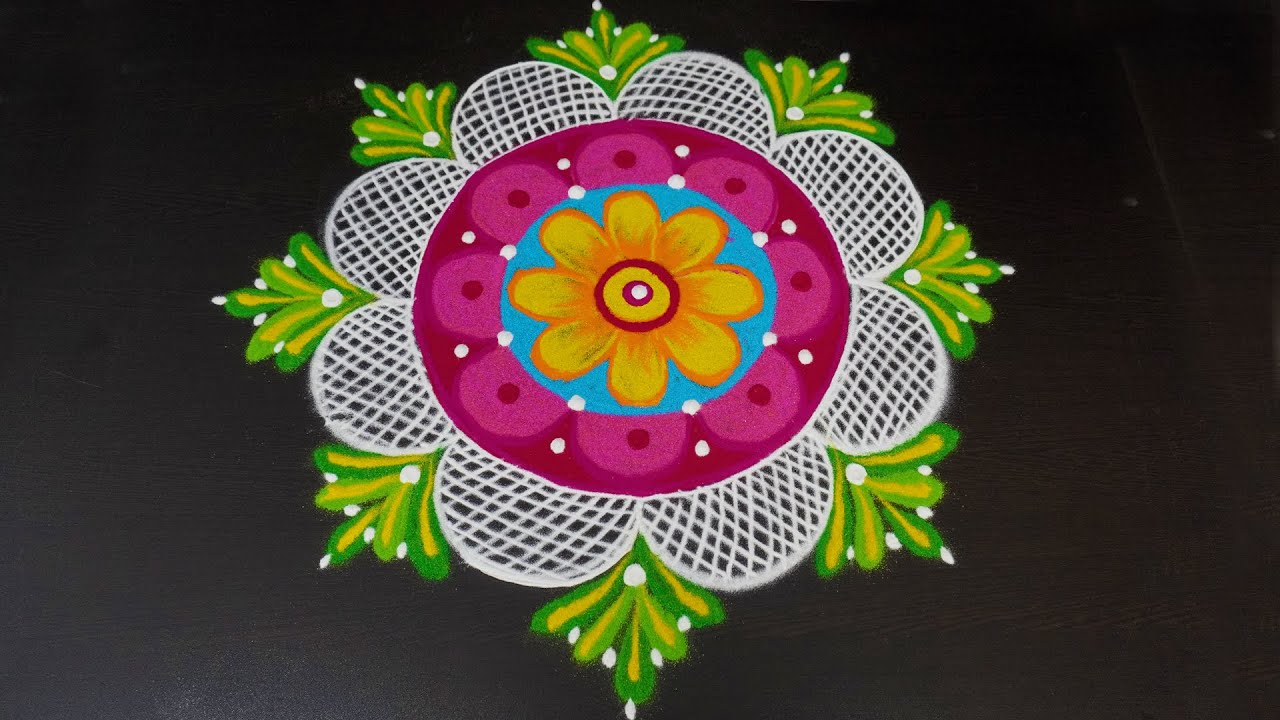Against a black background, this intricate piece of artwork resembles a flower, blending elements of embroidery and digital design. At the core, a white dot is enveloped by a red circle, followed by a yellow ring, another red circle, and then a yellow flower. The flower's petals exhibit two tones of yellow, with orange accents towards the center and outer edges. This floral motif sits atop a turquoise circle, which in turn is nestled within a dark pink circle adorned with lighter pink half circles and interspersing dark pink dots. Scattered white dots add further detail. Surrounding these central elements are large, white, mesh-like half circles suggesting flower petals, with green leaves—dark and light greens—protruding from each dip in the petals, resembling delicate, finger-like extensions or small trees.